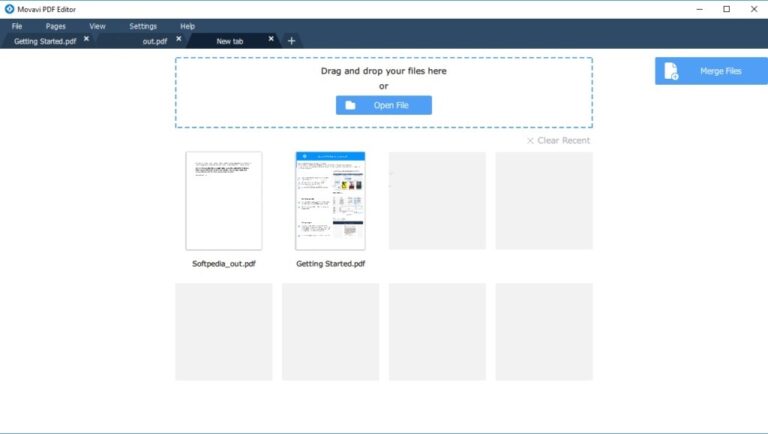This is a somewhat blurry screenshot of a computer screen, making the text difficult to discern. At the very top of the screen, a light blue horizontal line spans across the width. Directly beneath this is a horizontal white rectangle. In the upper right-hand corner, there is a blue circle containing a white symbol. Next to this circle is a word starting with the letter 'M', followed by the text "PDF Editor." Further to the right are the minimize, maximize, and close buttons.

Below this section lies a black rectangle with light-colored text in two rows on the left side, though the specific words are unreadable. Centered below this text, set against a white background, is a larger rectangle outlined with small blue dashes. Inside this outlined rectangle is a filled blue rectangle with a white file icon on the left side.

In the upper right-hand corner of this icon, there is another blue rectangle containing a white icon that appears to resemble a piece of paper, alongside the label "Merge Files" inscribed in white.

Centrally located on the screen are eight small gray square boxes arranged in a 4x2 grid. The first two squares on the top row feature document icons, while the remaining squares are plain gray.